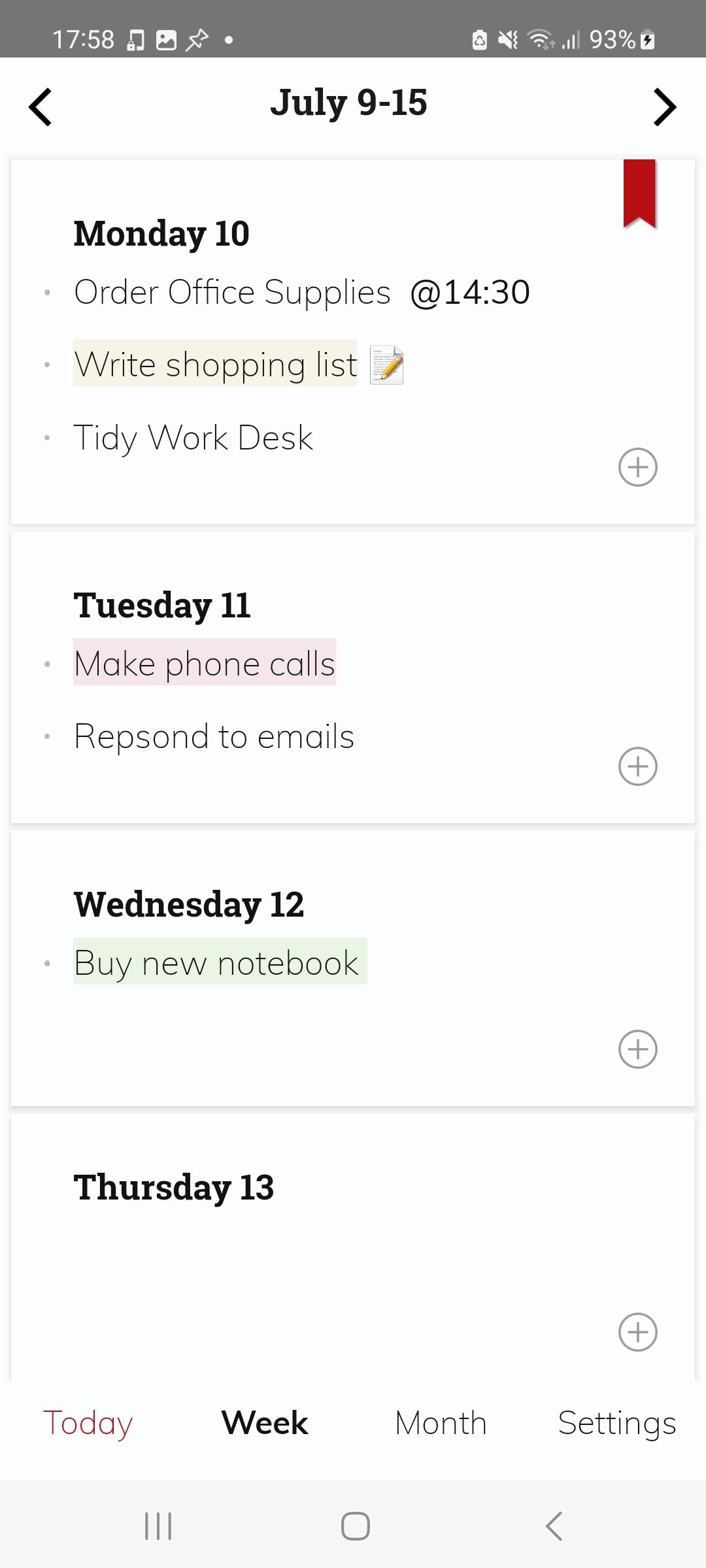The screenshot, captured from a smartphone, displays a detailed to-do list over a white background. The top header of the screen is a medium gray, signaling device status. On the right side of the header, icons show a battery at 93% with a black bolt indicating the phone is charging, Wi-Fi connectivity, and a muted phone symbolized by a line through a triangle. Additionally, another unidentified icon is present. On the left side, the time is shown as 17:58 in a 24-hour format, accompanied by more icons including a thumbtack and two squares.

Centered below the header on the white background, the date range is displayed in bold, dark gray font, reading "July 9 - 15." Flanking this date range are left and right arrows, and a vertical rectangle with a notched edge resembling a ribbon.

The to-do list entries are as follows:

**Monday 10**:
- Order office supplies at 14:30
- Write shopping list
- Tidy work desk

**Tuesday 11**:
- Make phone call (highlighted in light purple)
- Respond to emails (note: "respond" is misspelled as "repsond")

**Wednesday 12**:
- Buy new notebook (highlighted in gray)

**Thursday 13**:
- [No tasks listed]

The footer of the screen reads "Today," "Week" (bolded to indicate the current view), "Month," and "Settings."